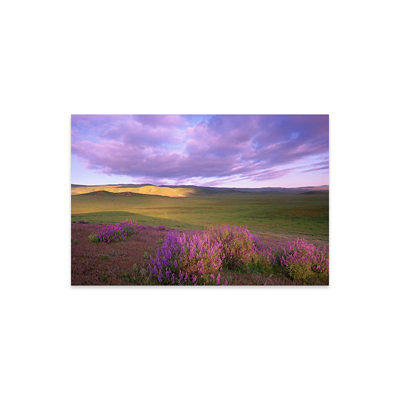The image depicts a small rectangular wall art mounted on a white background wall, showcasing a serene outdoor landscape that appears to be either a photograph or a painting. At the forefront of the image, vibrant lavender shrubs and tiny plants add a splash of purple to a wide, green grassy field with a few distinct bushes on the right. The setting is defined by gently rolling hills, illuminated by a warm beige glow in the center. The sky above features a mix of purple and blue hues, with clouds casting subtle shadows. The horizon is visible, transitioning from the grassy field to the cloud-strewn sky. Bathed in the bright light of a summer afternoon, the entire scene exudes a picturesque and tranquil atmosphere, capturing the beauty of nature in daylight without any text or additional markings.